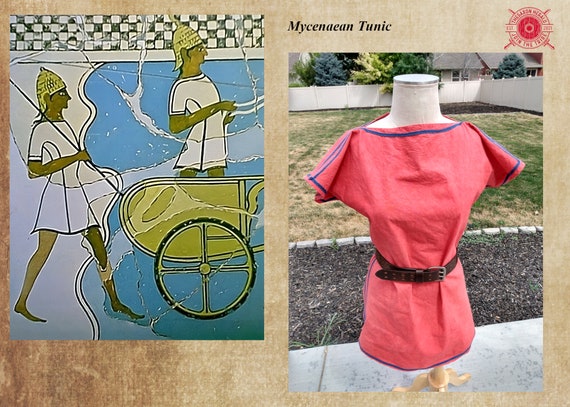The image features a beige-bordered composition of two pictures placed side-by-side. The left side showcases an artist’s rendition resembling ancient Egyptian times, depicting two barefoot men wearing white tunic-like clothing and gold hats. They appear staggered in their step, standing behind a half-visible gold carriage with a black wheel sporting four spokes. The background suggests a gathering of torn and reassembled paper, adding a textured effect.

The right side of the image presents a mannequin dressed in a pink tunic with purple piping and circled by a brown leather belt. This mannequin is placed outdoors, possibly in a yard, with visible grass, trees, and a white fence in the background. Above the mannequin, the text "Mycenaean Tunic" subtly integrates the historical theme between the two segments.